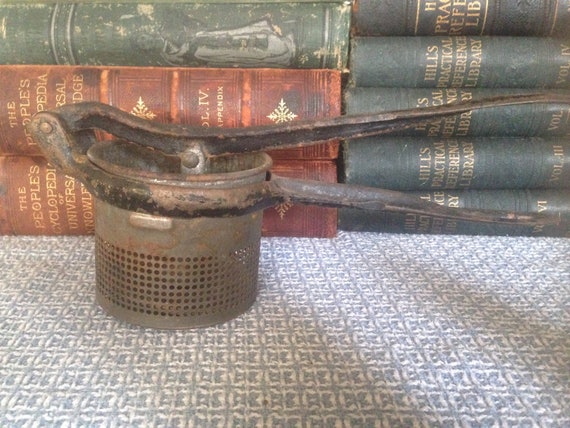The image depicts a detailed close-up of a mysterious and antique hand tool, appearing both worn and rusted, predominantly brown with blackish handles. The device is attached to a circular base perforated with holes reminiscent of a salt shaker, suggesting a specific, yet unclear, utility. Horizontally protruding handles extend from the center-right of the base, further enhancing its enigmatic nature. The background is composed of a neatly arranged assortment of books. On the left side, a set of three stacked gray-bound volumes, including "The People's Encyclopedia of Universal Knowledge" with visible gold-embossed titles. To the right, five books, possibly of the same series, are stacked with green bindings and covers, identified as "Hill's Practical Reference Library," also in gold lettering. The underlying surface is a checked tablecloth in brown, black, and white, adding a vintage ambiance to the scene. Natural lighting accentuates the clarity of the image, highlighting the contrasting textures and colors of the objects featured.